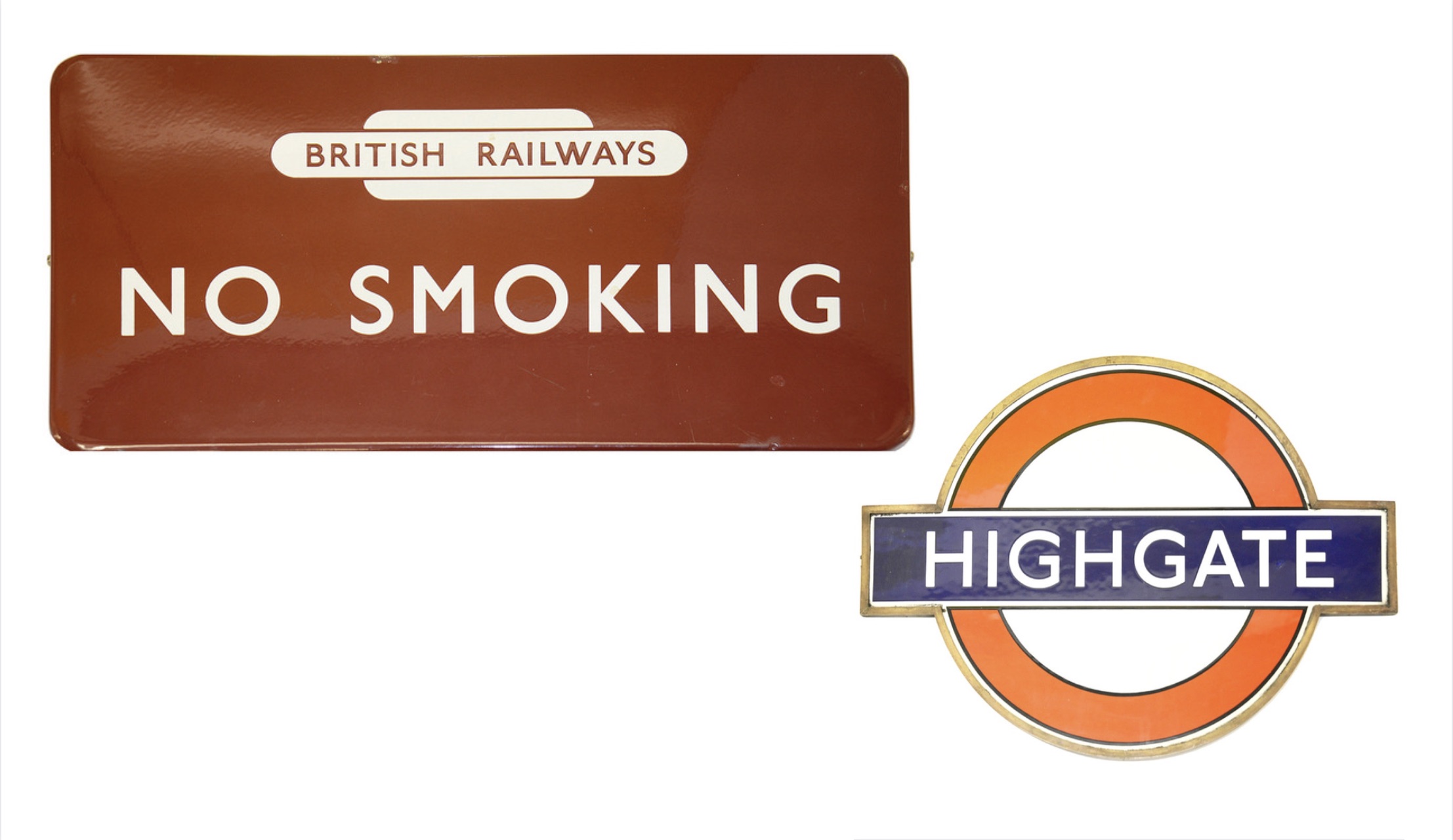This image showcases two distinct signs from a British railway station against a white background. On the left, a brown rectangular sign prominently displays the text "No Smoking" in bold white letters, with a smaller white banner above stating "British Railways." Slightly to the right and lower in position, there's a round emblem with an orange outline encircling a blue horizontal stripe. This stripe features the word "HIGHGATE" in all capitals, indicating Highgate tube station. Both items, seemingly pins or badges, are arranged side-by-side, creating a contrast against the white backdrop and suggesting a display of historical railway memorabilia.